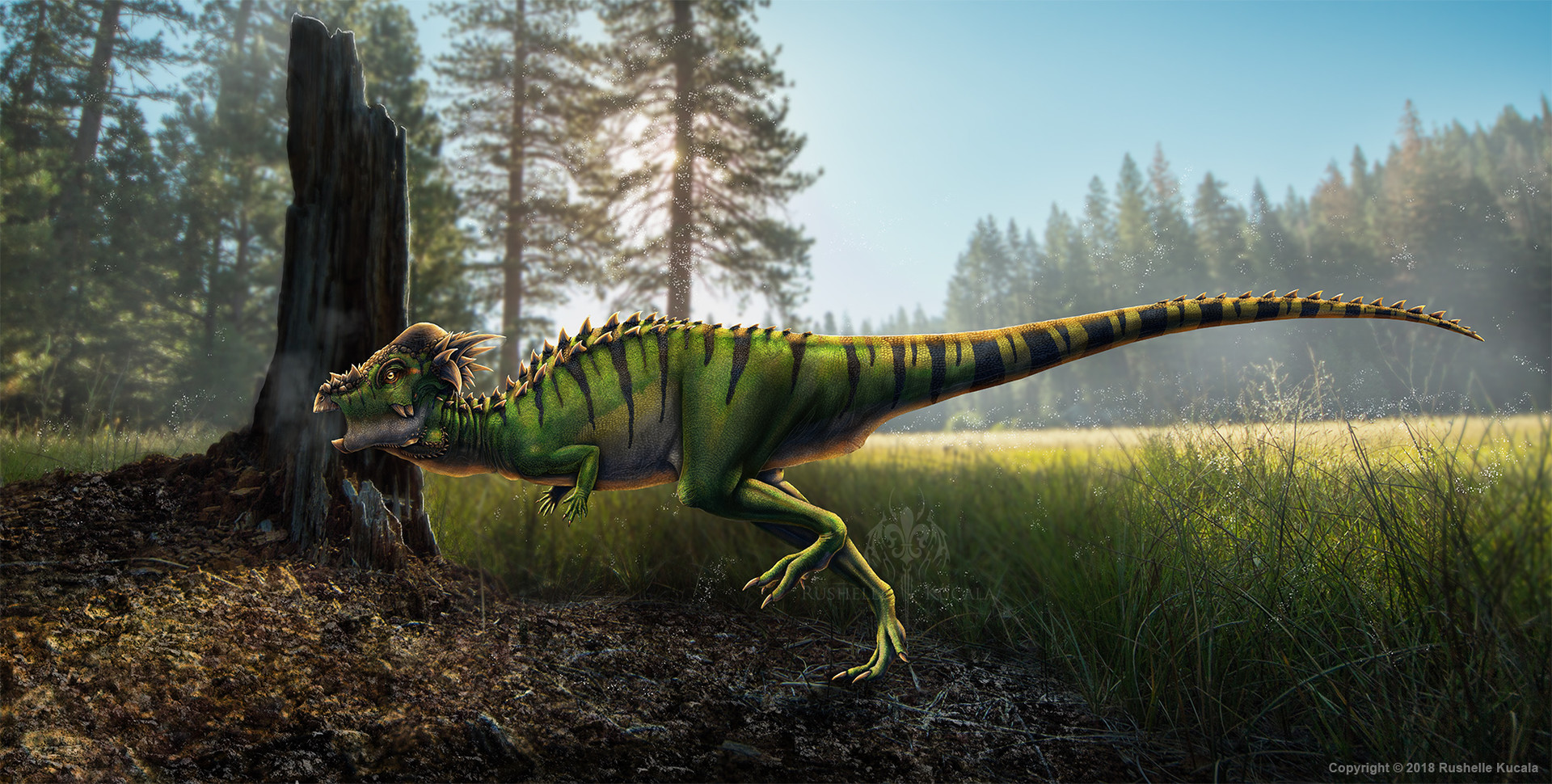The image is a detailed illustration of a small, green, raptor-like dinosaur with dark blue or black stripes running to the left. The dinosaur features a long tail adorned with short, spiky scales, small arms, and large legs, with its mouth open and yellow eyes peering forward. The background showcases a nature scene with a bright blue sky and sunlight filtering through green pine trees. In the foreground, there is bright green and yellow grass along with a broken tree stump slightly to the left of the dinosaur's head. Hints of early morning light permeate the scene, giving it a lifelike quality despite its likely AI-generated origin. The artwork is signed and dated "Rochelle 2018" at the bottom.